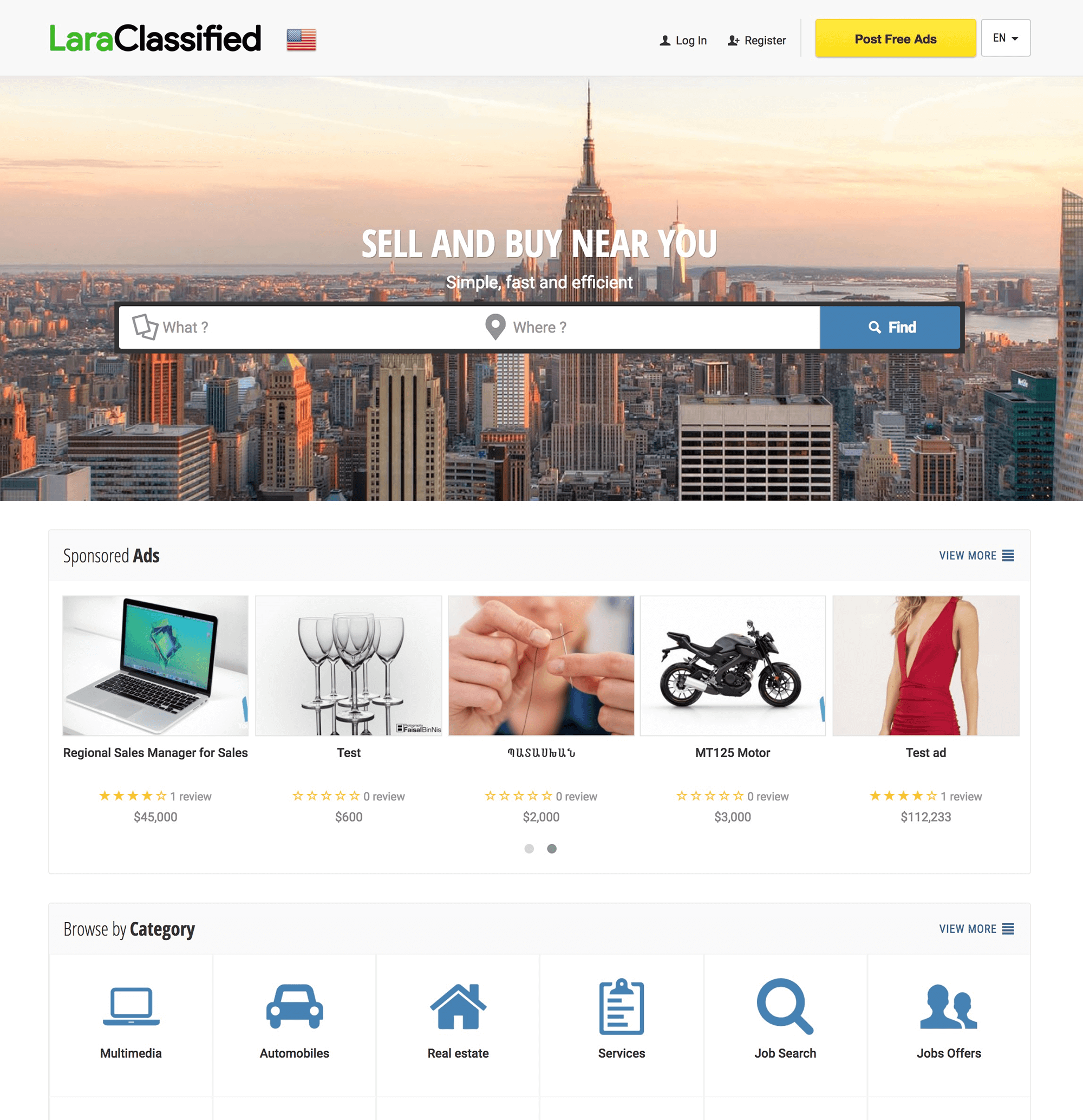The image depicts the Lara Classified website interface. In the upper left-hand corner, about two spaces to the right and one space down from the top, the text "Lara Classified" is displayed. "Lara" is in green with a capital 'L', and "Classified" is in black with a capital 'C'. The words are conjoined to appear as one. 

To the right of this text is an icon of the American flag. Following that, there is a right-aligned menu featuring the options "Login" and "Register". 

In its dedicated section, there is a yellow button with black text that reads "Post Free Ads". Next to it is a drop-down arrow within a white box that contains the Yen symbol in the middle. 

The main banner of the site showcases an aerial shot of a city's skyline, displaying the tops of various buildings. Centrally positioned on this banner are the words "Sell and Buy Near You". Below this text, smaller fonts spell out the site’s motto: "Simple. Fast. Efficient."

Directly beneath this tagline is a search bar, neatly integrated into the design for user convenience.